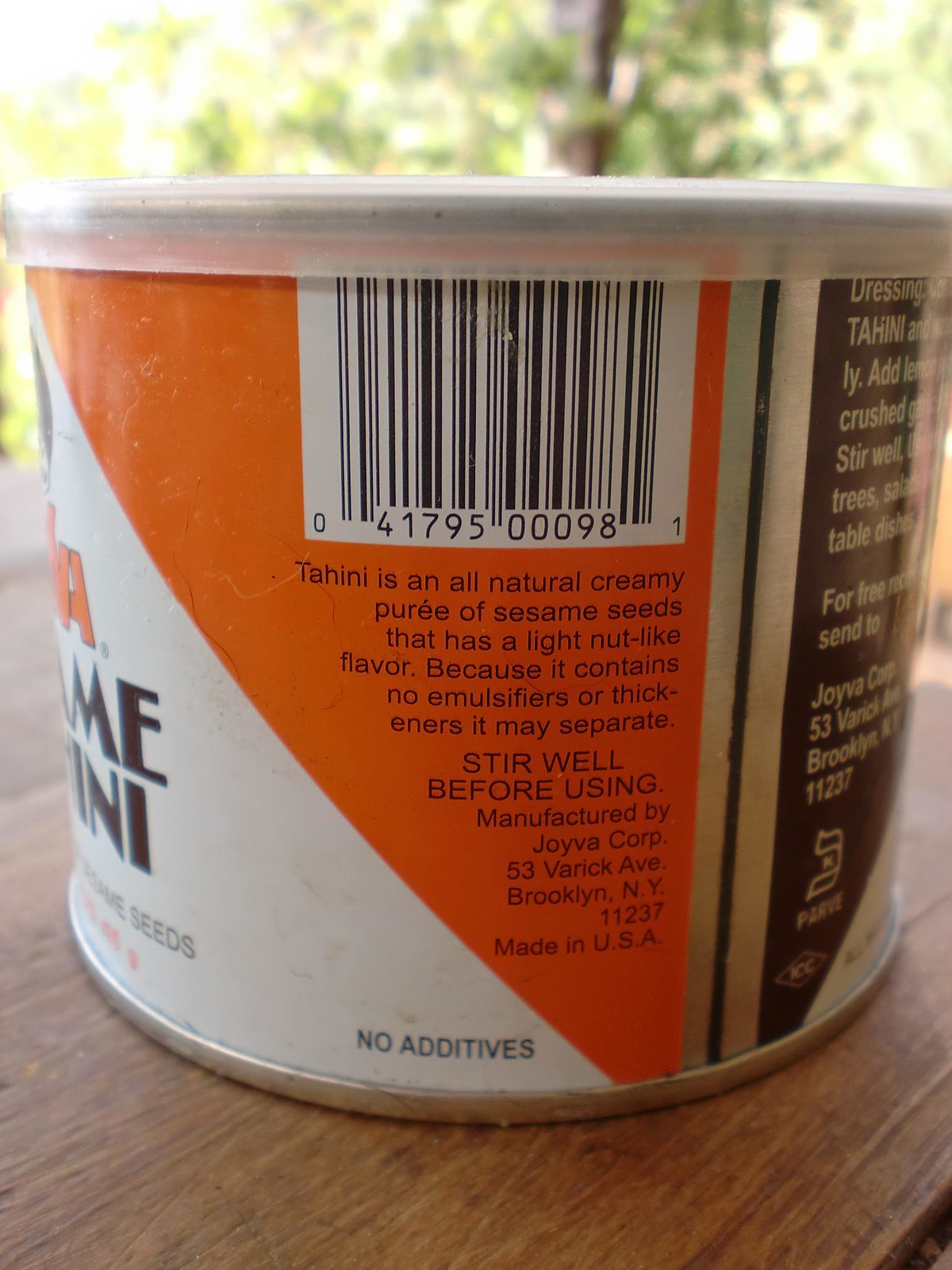Close-Up Image of a Tahini Canister with Detailed Label and Blurred Outdoor Background

The photograph captures a close-up view of a tahini product housed in a cylindrical canister. The visible side of the canister features a large orange triangle spanning the height of the container. Adjacent to the orange triangle, there's a white barcode with black lines and numbers reading "471950098," flanked by smaller numbers "0" and "1" on either side. Below the barcode, black text provides detailed information about the product: "Tahini is an all-natural creamy puree of sesame seeds that has a light nut-like flavor. Because it contains no emulsifiers or thickeners, it may separate. Stir well before using. Manufactured by Joyvecorp. 53 Variac Ave. Brooklyn and White. 11237. Made in USA."

The canister is topped with a clear plastic lid. To the right of the orange triangle, along the container's seam, is a section with a black background and white partial text, including words like "dressing," "tahini," "add," "crushed," "stir well," "trees," and "table" scattered in different rows. There's a small space indicating "free, send to," followed by the address again in white text alongside some manufacturing symbols and logos.

At the bottom of the orange triangle, the phrase "no additives" is displayed in black text on a white background that curves towards the front of the canister. The entire scene is set on a wooden table, with a blurred backdrop of green plants suggesting an outdoor environment.